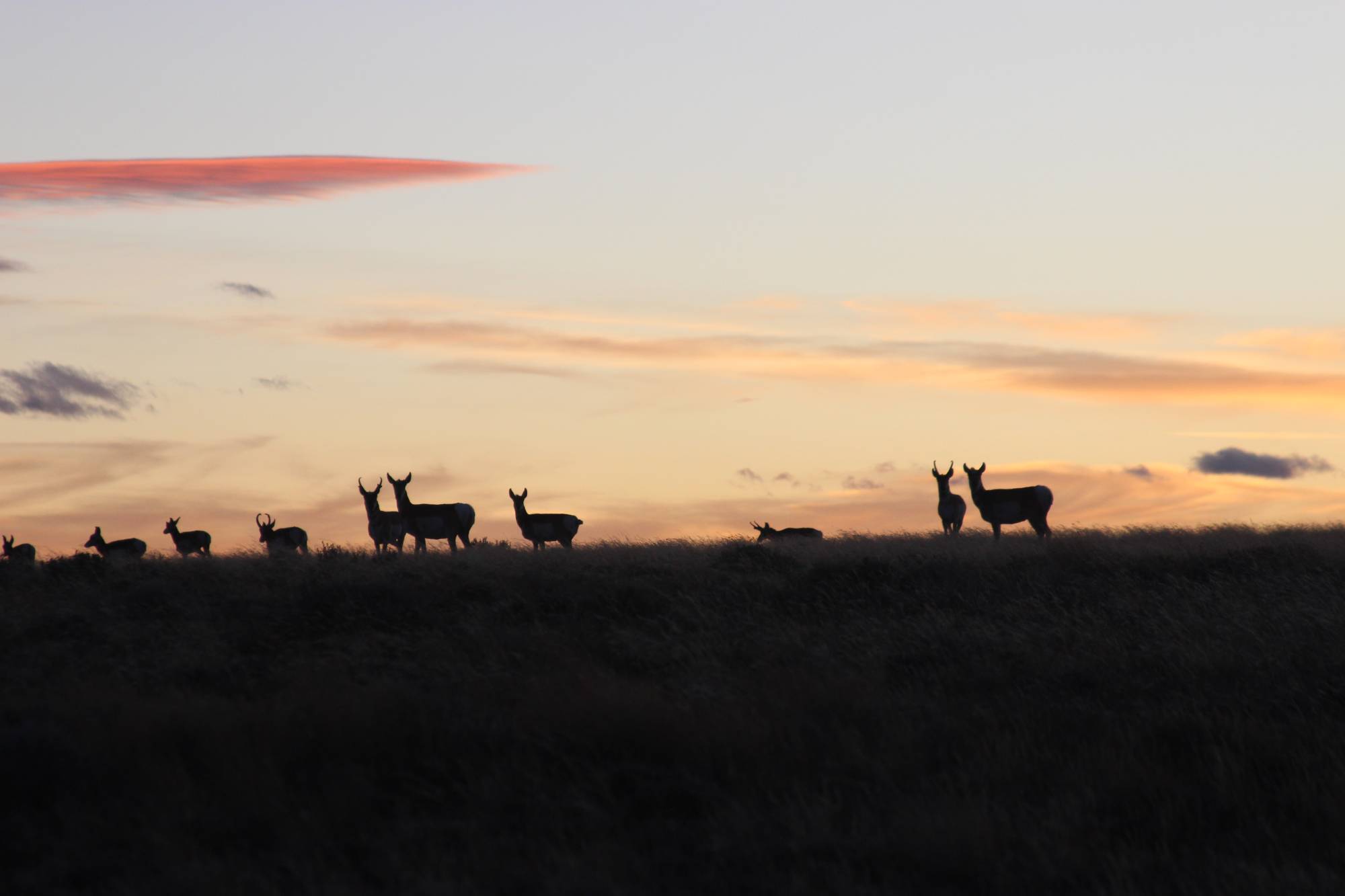In this captivating outdoor scene, the silhouettes of approximately 10 to 12 deer, varying in size and denoting males, females, and fawns, are beautifully framed against a vibrant sunrise or sunset sky. The deer are positioned atop a grassy hill, which, along with the ground, is rendered in deep shadow, allowing their dark forms to stand out starkly. The sky behind them is a breathtaking blend of creamy orange, peachy, blue, and gray hues, with one notably scarlet cloud adding a dramatic splash of color. The clouds scatter across the sky, contributing to the serene yet striking atmosphere. The deer appear in various poses—some standing attentively towards the horizon or the camera, while others rest on the ground—creating a natural, unsymmetrical arrangement that enhances the photo’s authenticity and charm.